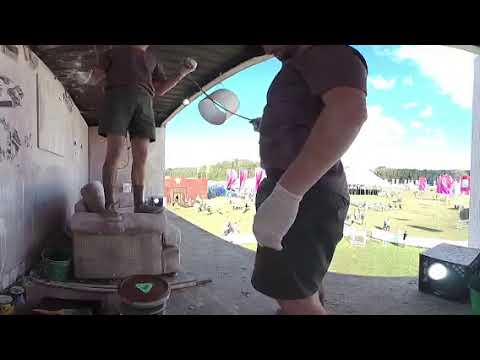This image captures two men engaged in construction work on the outside of what appears to be a house, specifically on a covered porch area. The photograph is vertically oriented, framed by black horizontal stripes at the top and bottom. Both men are dressed in identical uniforms consisting of brown t-shirts, dark green or gray shorts, white gloves, mid-calf black socks, and dark shoes. One man stands on the arm of a dirty, old white couch, elevating himself to work on the ceiling. He holds a cord with a white open cylinder or lampshade attached, suggesting they might be installing a ceiling light. The second man, positioned closer to the camera, grips a metal rod with a similarly attached white cylinder. The porch floor and wall are made of gray concrete, and a dark brown crate is visible behind the men alongside various colored buckets and painting supplies, including a paintbrush in a flat tray. Beyond the porch, the scene opens up to a green lawn strewn with numerous objects, such as porta-johns, tents, and appliances, adding to the construction site atmosphere. The covered ceiling above them is dark brown, while the open area behind reveals trees and more greenery.